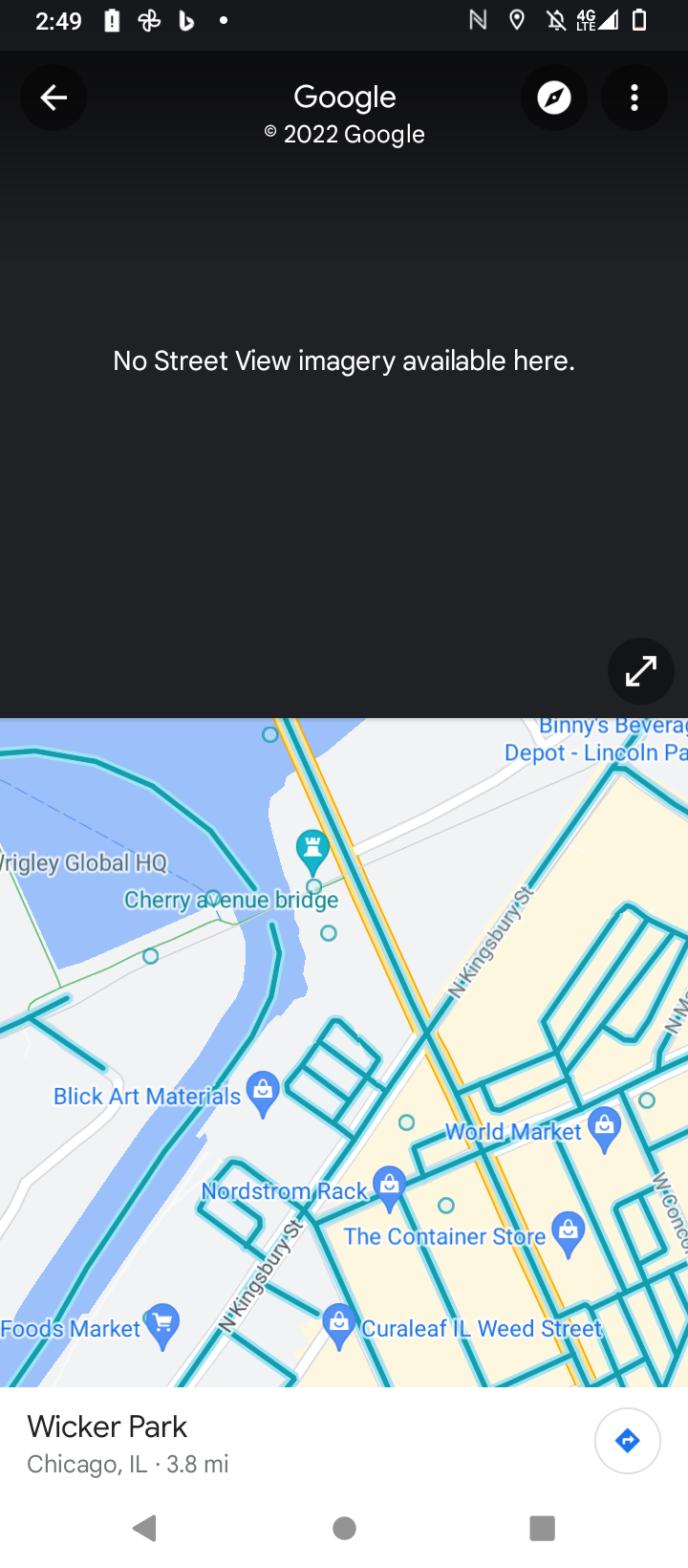This is a screenshot captured from my cell phone. At the top, the notification bar is visible, indicating the time as 2:49. The battery icon is displayed alongside the 4G LTE signal strength indicator and a muted sound icon, evidenced by a line through a speaker symbol. Additionally, the GPS icon and several other notification symbols are present.

Dominating the screenshot is a black box resembling a dropdown from an app, marked "Google 2022 Google." Centrally within this box, the message "No Street View imagery available here." is displayed. Below this black box, a portion of a map, likely from a GPS or map application, is visible, providing a contextual backdrop to the information above.